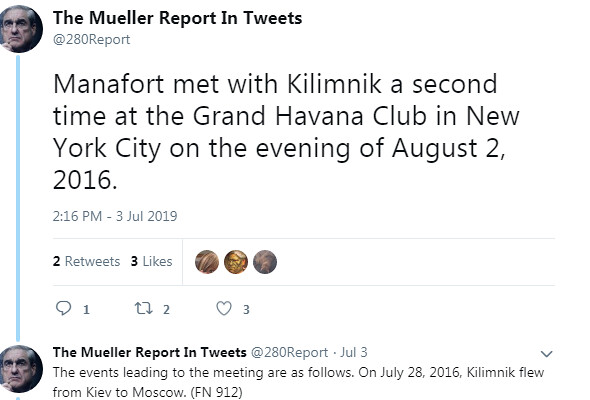The image is a landscape-oriented social media post resembling a screenshot from Twitter, featuring a photograph of Robert Mueller on the top left. Adjacent to the photo, the account name is labeled "The Mueller Report and Tweets" with the handle @280Report. The main tweet states: "Manafort met with Kilimnik a second time at the Grand Havana Club in New York City on the evening of August 2, 2016." This tweet was posted at 2:16 p.m. on July 3, 2019, and garnered two retweets and three likes. Below this tweet, the same account commented on July 3, 2019, with: "The events leading to the meeting are as follows. On July 28, 2016, Kilimnik flew from Kyiv to Moscow (FN-912)." A blue vertical line visually connects the original tweet and the comment, emphasizing the linkage. Notably, the account lacks a verified blue checkmark, making the source of the information uncertain.